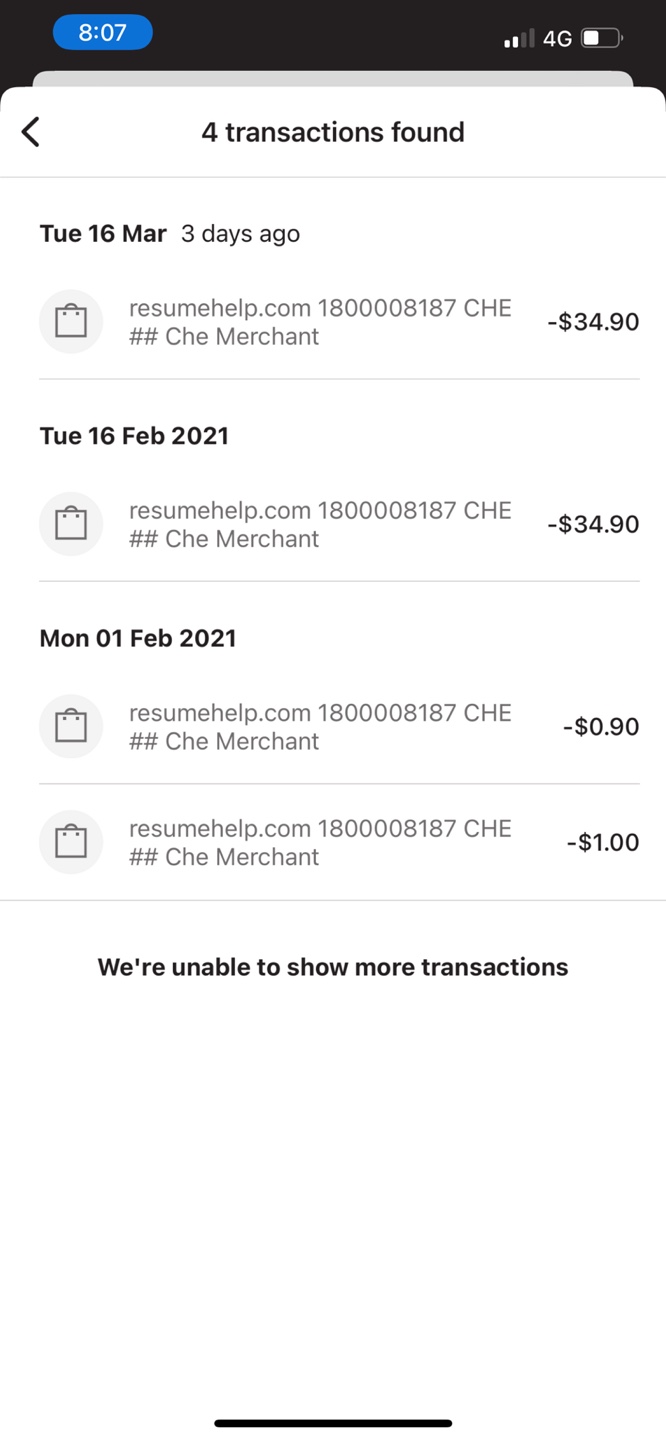This is a detailed screenshot of a smartphone display showing a series of financial transactions, presumably from a bank account or credit card statement. The top of the screen has a horizontal black border. In the upper left-hand corner, inside a red or blue oval, the time is displayed as 8:07. The upper right-hand corner shows the device status with two bars of signal strength, a 4G network indicator, and a half-full battery icon.

Below this border, the screen background is white, with a header that reads "4 transactions found." 

The transaction details are listed as follows:
- Tuesday, March 16: A payment to resumehelp.com for $34.90.
- Tuesday, February 16, 2021: Another payment to resumehelp.com for $34.90.
- Monday, February 1, 2021: Two separate transactions from resumehelp.com, one for $0.90 and another for $1.00.

At the bottom center of the screen, there is a message that states, "We're unable to show more transactions."